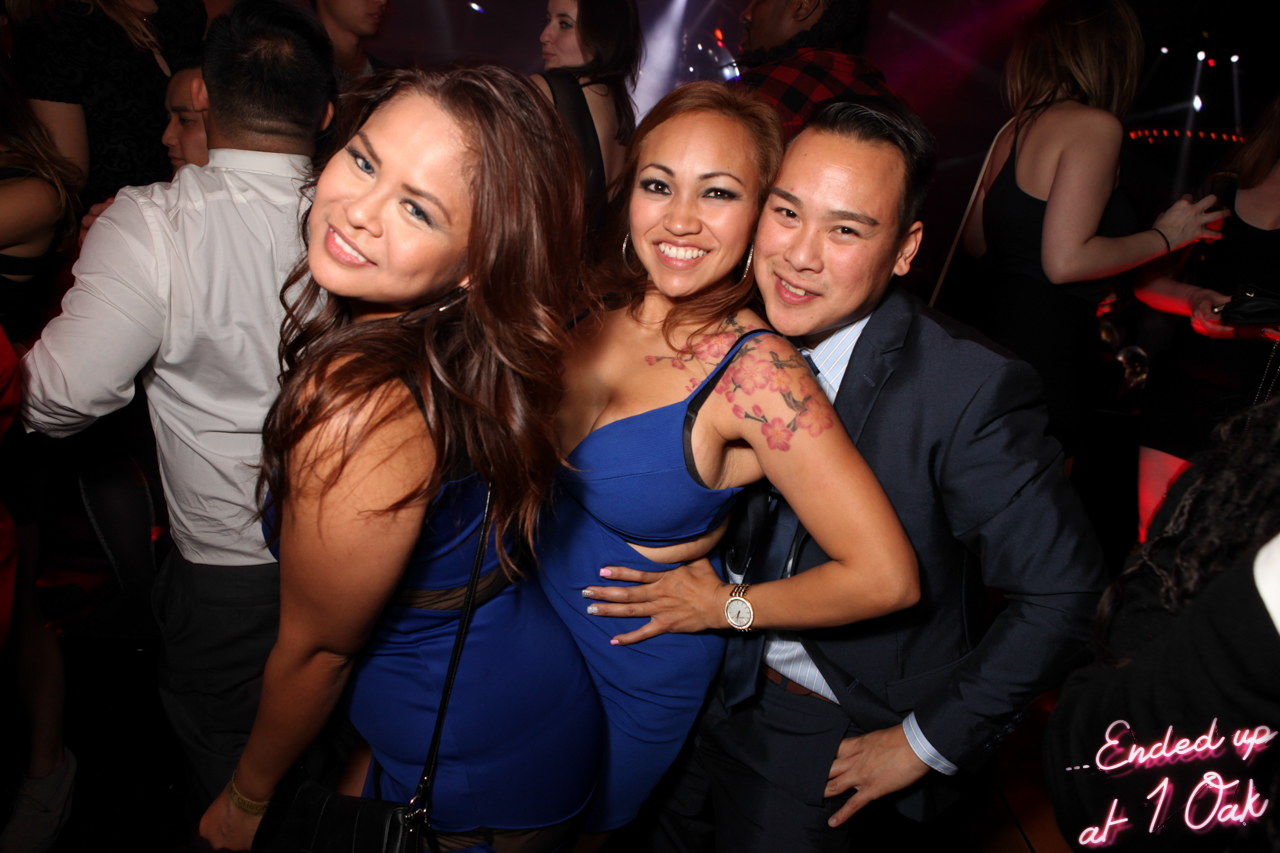In a vibrant nightclub scene, the main focus of the photo is on three young Asian partygoers, all exuding energy and joy. Centered in the shot is a pretty young woman, likely between 20 and 25 years old, with long, wavy, dark brunette hair cascading over her shoulders, adorned in a form-fitting, royal blue dress. She's smiling seductively at the camera, her left arm relaxed by her side, and a wristwatch with a white interface glimmers on her wrist. To her right, a girl with slightly reddish-brown hair, also in a tight, low-cut blue dress, is showing off a striking tattoo of Japanese cherry blossoms on her upper arm and shoulder. She is smiling broadly, clearly enjoying the moment, and is being embraced closely by a man. This man, with short black hair, is dressed sharply in a dark suit jacket, white collared shirt, and a dark blue tie. They're all clearly reveling in the lively atmosphere, with the background revealing more partygoers—some dancing, others chatting. In the bottom right corner of the image, in stylish pink cursive and white lettering, it reads, "ended up at one oak."